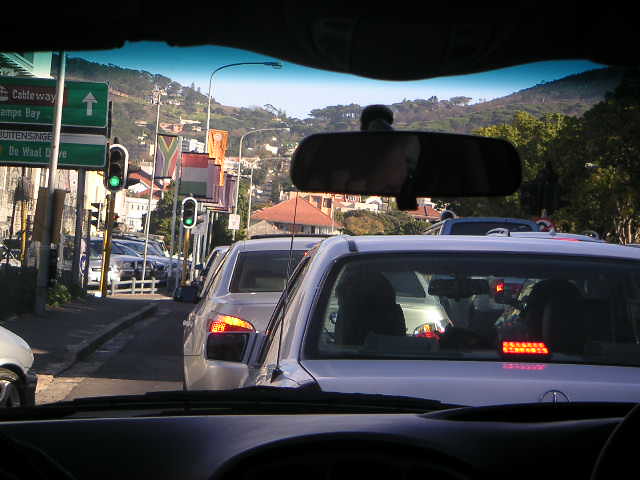A photograph captures a bumper-to-bumper traffic jam, seen from inside a car looking forward. The car’s dark rearview mirror is visible but indistinct. To the left, a car is attempting to merge into the lane. Ahead, an array of brake lights are illuminated, indicating the standstill congestion. Directly in front, a Mercedes is prominently displayed, with its emblem discernible and a person visible within. In the distance, a city sprawls over hilly terrain, adorned with greenery and trees. One notable building features a red slate roof. Despite multiple green traffic lights in sight, the traffic remains immobile. Light poles are also scattered throughout the scene. It is daytime, as evidenced by the clarity of the surroundings, and a green directional sign looms ahead, although progress is halted.